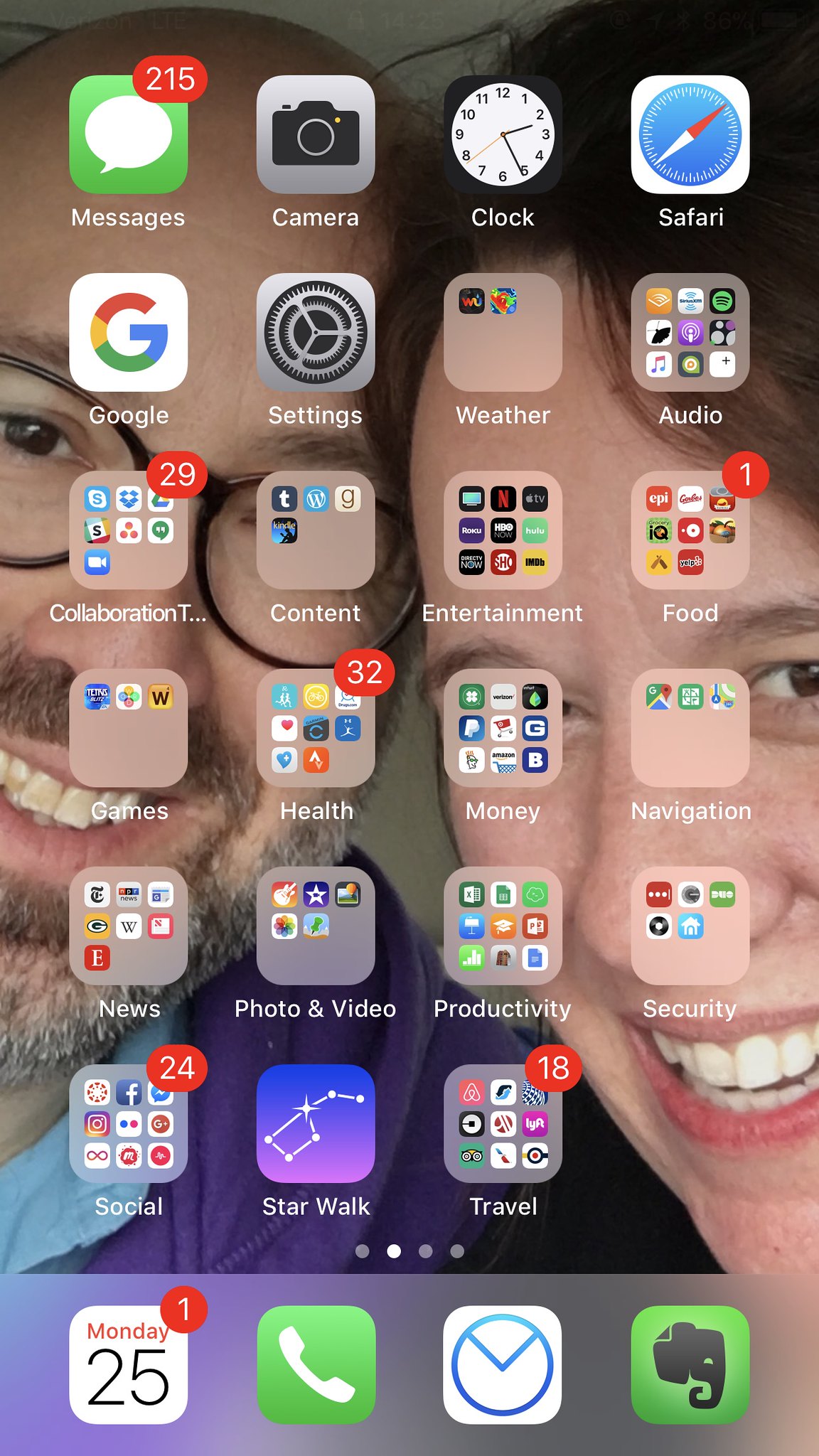This detailed screenshot captures an iPhone home screen, featuring a personal background image of two smiling individuals with their heads close together. Both appear to be Caucasian. The man on the left sports a short beard, black glasses, and a purple sweatshirt, while the woman on the right has long black hair, and her attire is not visible. 

The home screen showcases various app icons, some with notification badges. In the top left corner sits the Messages app, easily identifiable by its green square and white text bubble, prominently displaying a red notification badge with the number 215, indicating unread messages. The screen also contains several folders, some with red badges signaling unread notifications, while others remain badge-free. 

Additionally, there are individual apps without any notification indicators. At the bottom of the screen, four dots suggest that this is just one of multiple pages of apps, hinting at the possibility of swiping left or right to explore more.